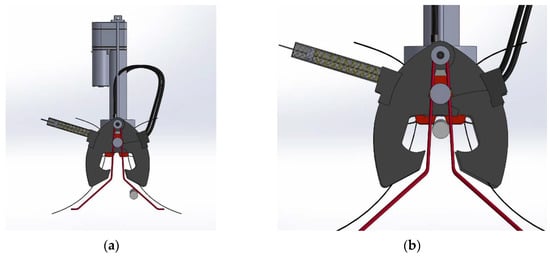In this photograph, we see two images that display different perspectives of the same futuristic helmet. The image on the right provides an up-close view of the helmet, showcasing intricate features such as slits for the eyes, nose, and mouth. The left side of the helmet displays a protruding elongated stick with a spike at the end, while a small electric cable is visible on the right side, plugging into the helmet. Red lines run from the top to the bottom of the helmet, adding a striking detail.

The image on the left offers a more expanded view, allowing us to see additional features that were not visible in the close-up shot. The electric cable on the right side can be traced as it connects to the back of the helmet. Behind the helmet, a tall, silverish metallic object is visible, suggesting some kind of dispensing mechanism, though its specific function remains unclear. This detailed depiction highlights the complexity and futuristic design of the helmet.